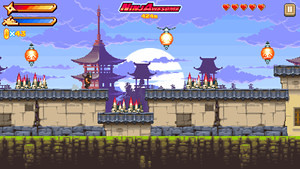The image appears to be a screenshot from a video game, framed in a horizontal rectangle. At the top of the screen, there is a prominent gold bar, followed by a smaller gold bar adorned with a four-pointed star. Directly beneath these, a blue bar is displayed. Centered within these bars is text, blurry but seemingly reading "NINJ NINJA Ninja," and possibly "AWESOME" thereafter.

Below this text are five red hearts, indicating a health or life meter. Further details include a hard-to-read gold number, potentially "424-something," situated under "NINJA AWESOME." Moving to the left at the top of the screen, there is a gold zero followed by an "X" and the number "43" in gold, likely representing a score or item count.

Visually, the scene is set in an Asian-inspired environment. A stucco-like wall cuts through the middle of the image, flanked by two traditional Asian buildings with distinctive roofs that swoop downwards and curl up at the edges. The sky above is blue with a hint of blue-violet in the clouds, contributing to the overall atmosphere. The left building features dark pink shadows, adding to the depth and color contrast. Below the stucco roof, the wall is beige, resembling large stone, while the lower section transitions into a blue wall bordered by green bushes at the bottom.